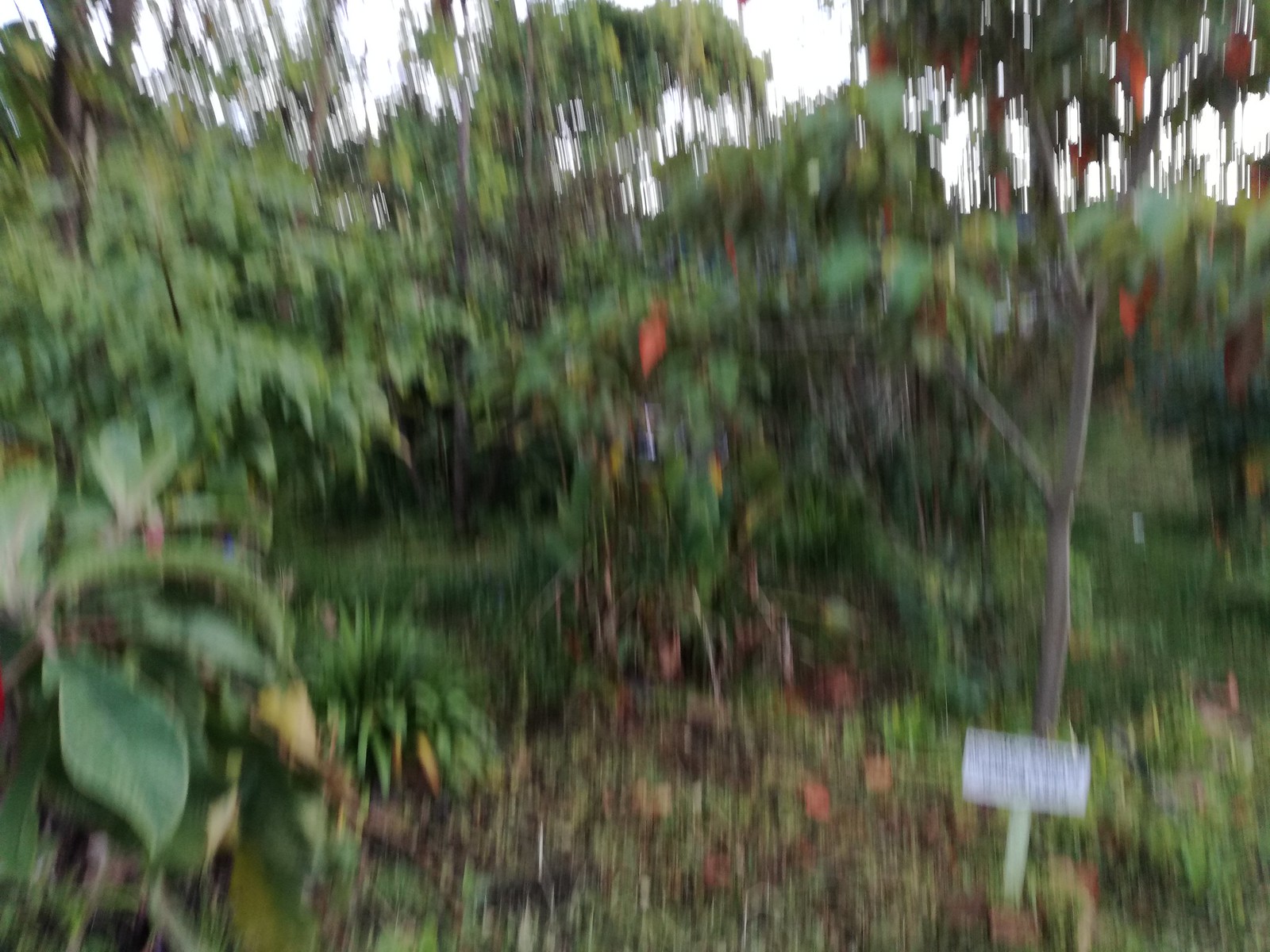The photograph, taken outdoors, is a color image captured during the daytime in landscape format. Despite its extreme blurriness and low resolution, several details emerge. In the background, there are larger trees, some of which resemble weeping willows, with patches of whitish-gray sky visible through their foliage. Coming closer to the foreground, the vegetation thickens with various bushes and plants featuring a mix of pointy and smooth, teardrop-shaped leaves. Among them, some plants bear red leaves, and others appear to have what look like peppers hanging from their branches, suggesting a well-maintained, healthy green field or orchard scene. Prominently, in the right-hand corner, stands a skinny, tall tree with a white rectangular sign affixed to its trunk, although the writing on the sign is illegible. The foreground features a grassy area, adding to the lush, tropical ambiance of the setting.